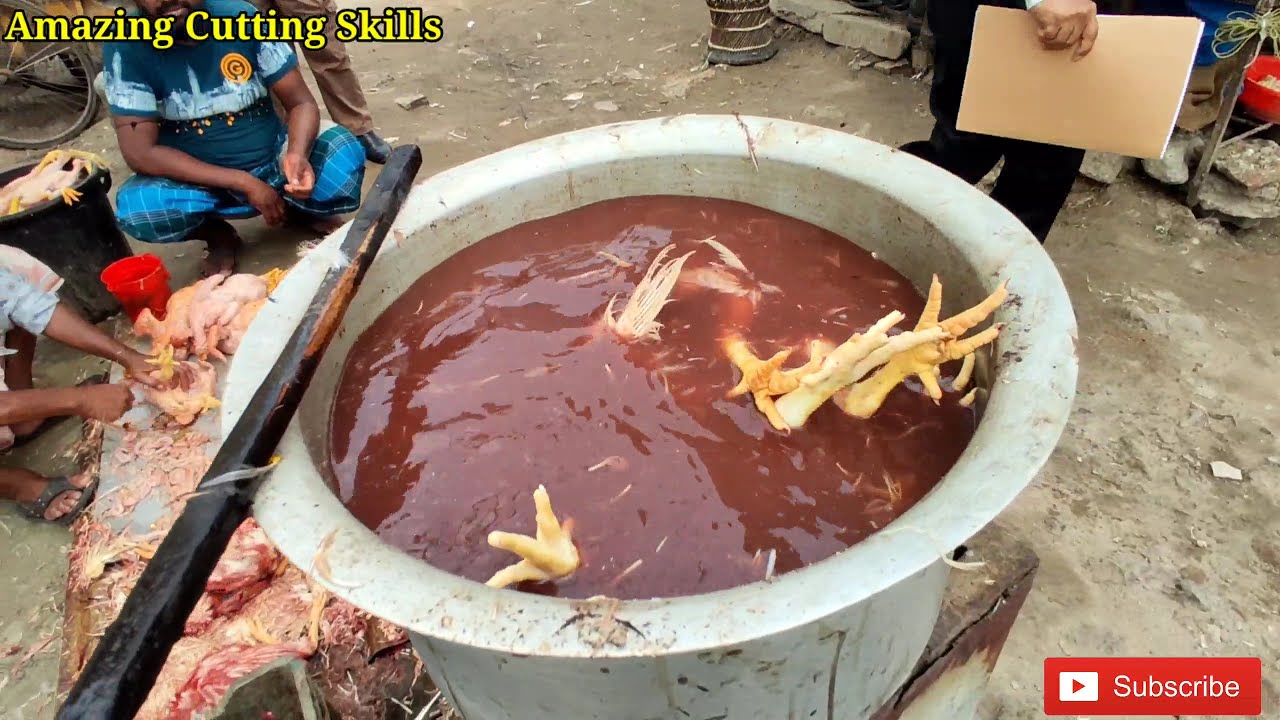The image, a screenshot from a YouTube video, is a vivid and slightly unsettling scene centered around a massive, round metal pot filled to the brim with a dark red, almost crimson liquid. Floating conspicuously within the pot are numerous bright yellow chicken feet, some partially visible, making for a striking and somewhat disturbing visual. Positioned prominently at the very bottom right corner of the image is the red YouTube subscribe button with the iconic play symbol, indicating the platform's affiliation.

The pot, situated outdoors on a primitive and unsanitary stone base amidst a dirt floor strewn with rocks, dominates the center of the image. To the bottom left, two men are actively engaged in preparing dead chickens on a makeshift board. One man, clearly visible, wears a dark blue soccer jersey adorned with a yellow G logo, suggesting an Indian or Middle Eastern ethnicity. Surrounding them, feathers, bits of muscle meat, and blood contribute to an overall sense of disarray and lack of cleanliness. In the background, a man carrying a manila envelope strides from left to right, though only his black pants are mostly visible.

A black metal rod, possibly used for stirring, lies across the pot, further accentuating the scene's rudimentary nature. At the top left of the image, the yellow text "Amazing Cutting Skills" is prominently displayed as a watermark. The chaotic and rustic setting amplifies the third-world country ambiance, illustrating a raw look at food preparation in less sanitized environments.